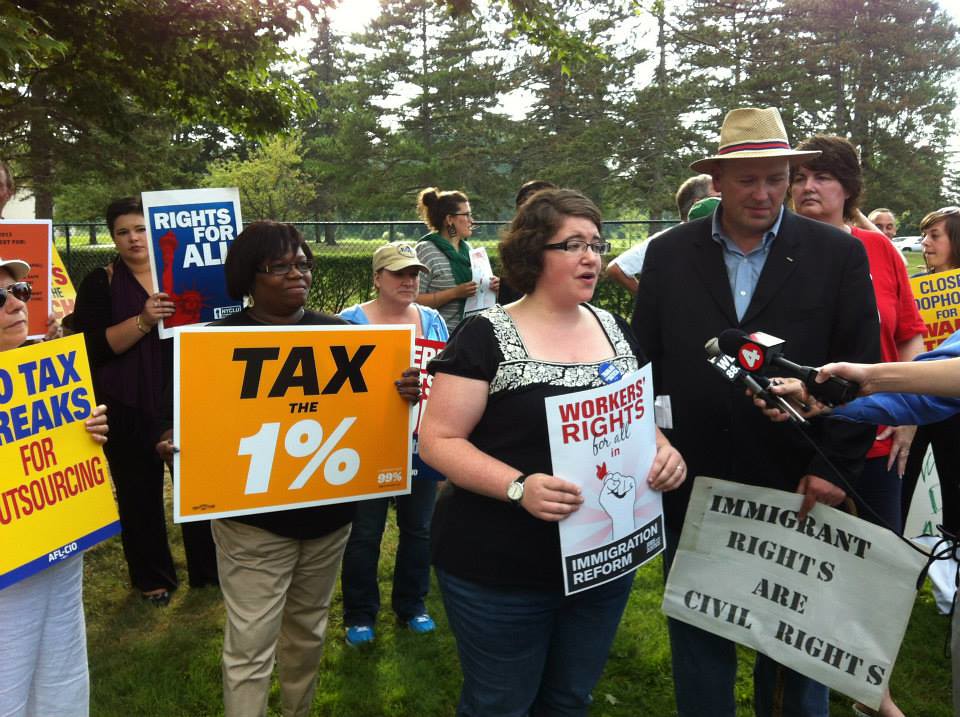In a sunlit, grassy park, a diverse group of protesters has gathered, many holding up various colorful signs advocating for different causes. Standing prominently on the right side, a man in a black suit with a blue shirt and a straw hat is being interviewed by reporters, with two microphones pointed towards him—one marked with a red square and the number four, and the other partially obscured showing only the letter 'W'. His sign remains lowered, almost hidden. 

Next to him, a woman with short, dark hair and black glasses wears a black shirt with white trim and blue jeans, and she is holding a sign that reads "Workers' Rights for All" above a white fist grasping a red object. Below are the words "Immigration Reform" against a black background. To her left stands a black woman in khaki pants and a black shirt, holding a bright orange sign saying "Tax the 1%". 

In the background, another protester holds a sign stating "Rights for All", set against a backdrop of lush green trees and a chain-link fence that stretches to the height of the protesters' heads. Through the leafy canopy, hazy sunlight filters across the scene, illuminating the fervent collection of signs, contrasting colors, and passionate expressions of advocacy for rights and reforms.